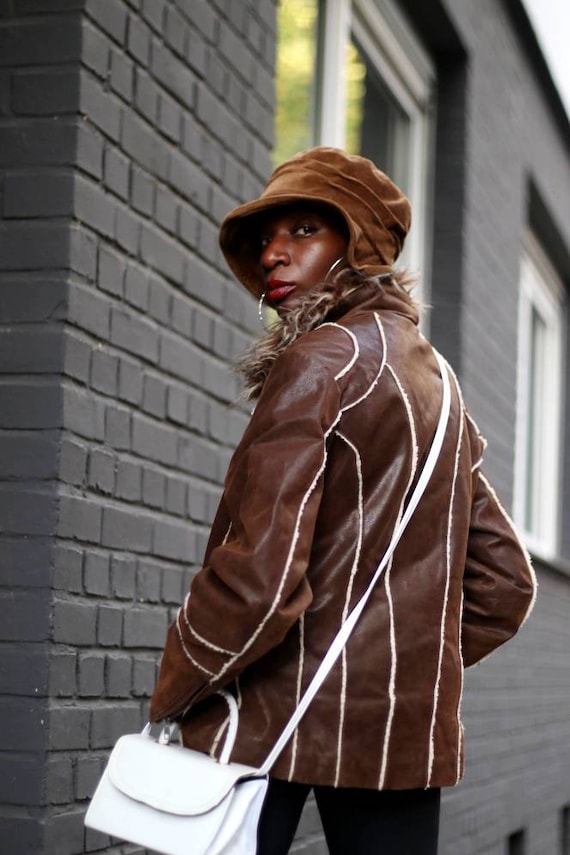The image features a stylish black woman walking down the street in front of a gray brick building with two white-framed windows. She is wearing a chic brown leather jacket adorned with thin white stripes and a brown hat pulled low over her head, partially obscuring her face. Her striking silver hoop earrings and a small white pocketbook, slung across her shoulder to the front left, add to her fashionable appearance. The woman, who exudes a model-like aura, has her back towards the camera but is looking over her left shoulder, capturing her expressive eyes and closed lips. The building also features two smaller, basement-level windows, providing a nuanced architectural backdrop to this evocative urban scene.